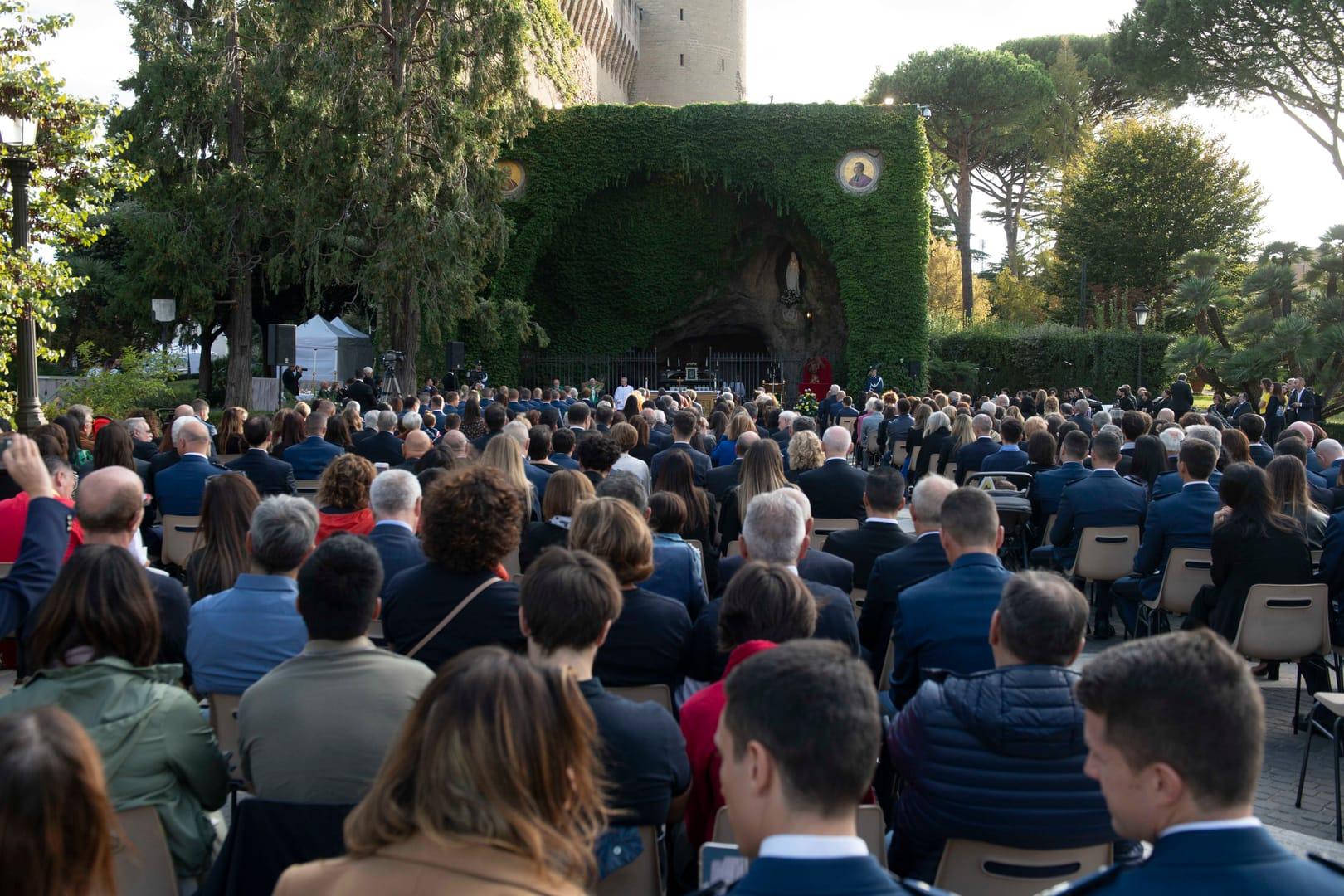The image captures a large outdoor gathering where a diverse crowd of men, women, elderly, and boys are seated in multiple rows of chairs, all facing towards a stage or pulpit adorned with a green arch. The bottom of the frame focuses on the backs of four individuals' heads, with the rows extending back and widening to about eight or ten people across. Attendees are dressed in a variety of colorful coats, including navy blue, brown, and red. The right side of the image features an aisle separating two sections of seating. The stage area, located in the upper middle part of the image, is flanked by greenery, with trees to the left and hedges to the right, extending to more trees. Beyond this stage in the background, a building is faintly visible, completing the serene, natural atmosphere of the event.